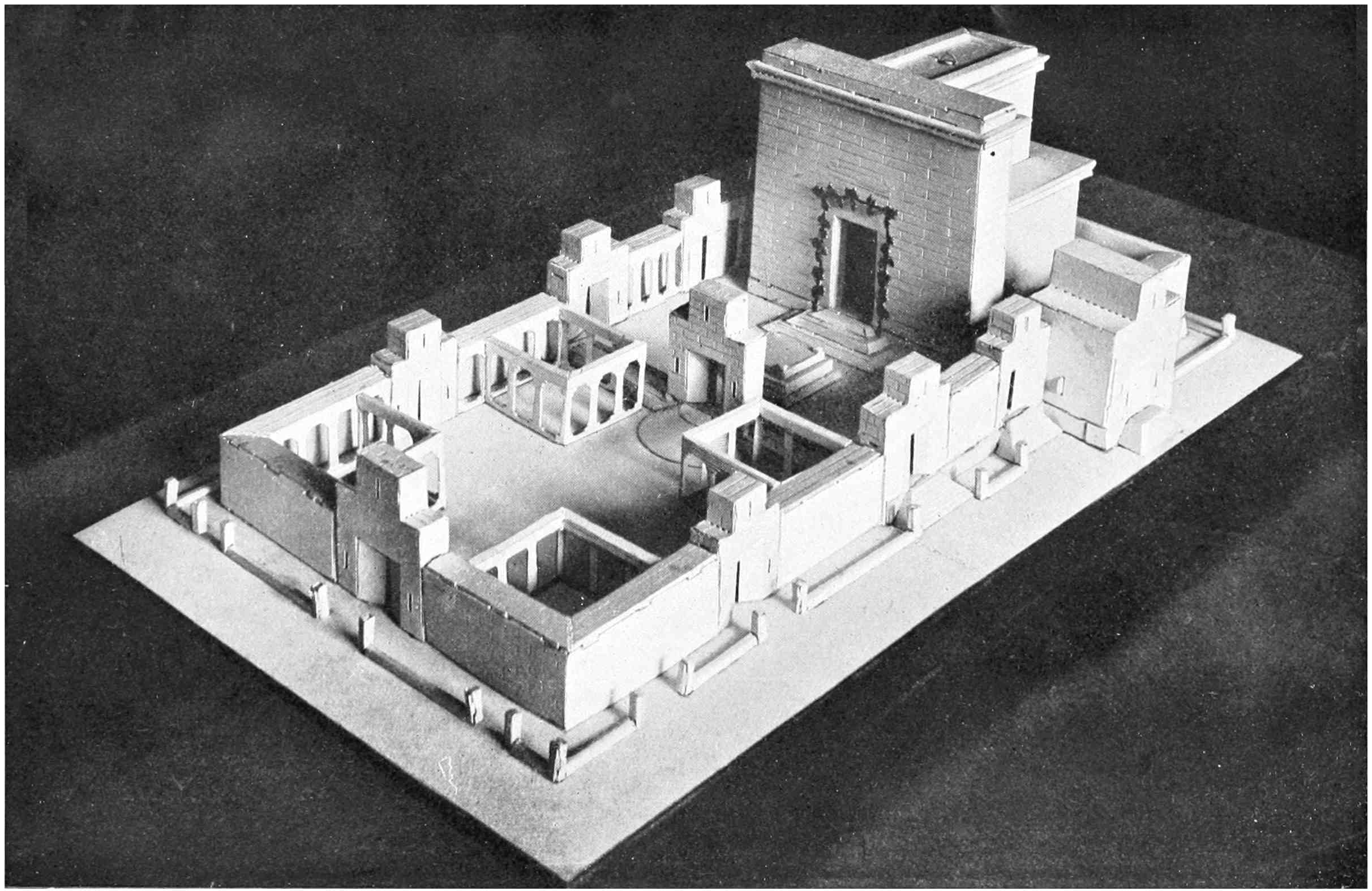This black and white photograph captures a detailed three-dimensional diorama of an ancient temple complex. The intricately crafted model appears to be made primarily from clay, accented with wooden pieces, and likely rests on a black table with a black backdrop, enhancing its contrast and detail. The main feature is a central temple with garlands adorning the entrance. This central structure is accessed through a series of gates and multiple rooms branching off from the sides. In front of the temple is a courtyard defined by thick, rectangular walls with distinctive square protrusions at the top. A smaller gate precedes the main temple entrance, leading into the courtyard, which contains four sub-areas marked by walls. The background of the scene is completely dark, making it difficult to discern finer details like the possible color of the model, though it appears to be white or yellow in parts. Vines and foliage are suggested to be growing around some of the doors, adding to the ancient and well-worn appearance of the complex. Despite the numerous details, the specific period and the civilization it represents remain unidentified, maintaining an air of mystery around the diorama.